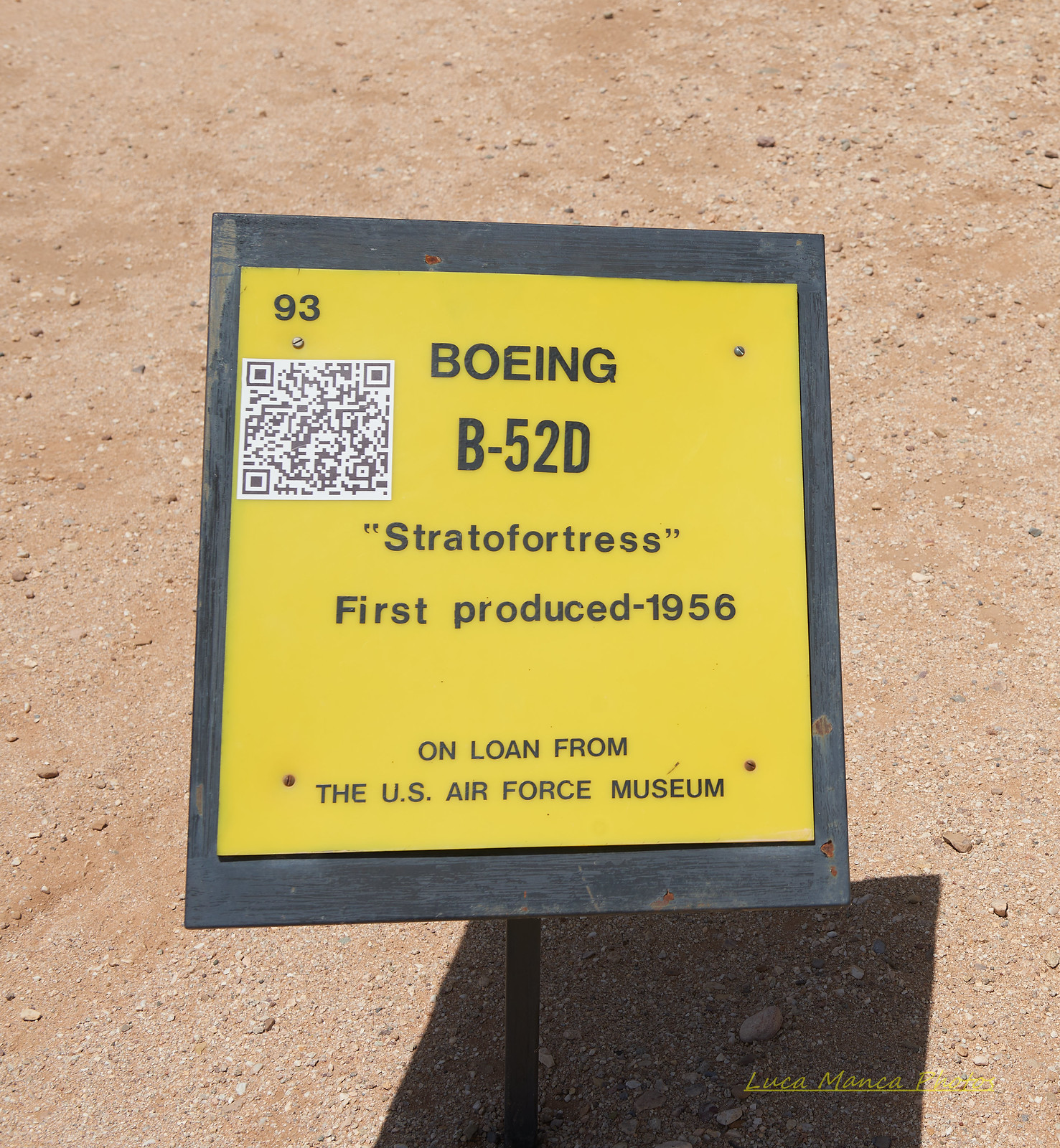The image depicts an outdoor exhibit of an aircraft, likely at an airplane museum or graveyard. The background is primarily sandy or gray, indicating a dirt field under the bright sun, as evidenced by the shadow of the sign cast beneath it. The focal point of the image is a substantial, sturdy metal signpost with a black wooden background, designed to provide detailed information about the aircraft, although no actual jets or airplanes are visible in the image.

The sign is square with a prominent yellow, likely plastic, section bolted to it. At the top left corner, the number "93" is displayed in black. Directly below this, a QR code is positioned for scanning to acquire more information. The main body of the sign reads "Boeing B-52D" in large, black letters on the yellow background. Beneath this, in smaller uppercase letters within quotation marks, it states "Stratofortress." Further down on the sign, it specifies "First produced: 1956," followed by the statement "On loan from the U.S. Air Force Museum" at the bottom.

This sign, typical for aircraft exhibitions, provides essential historical details about the Boeing B-52D Stratofortress and stands prominently to educate visitors about its significance.